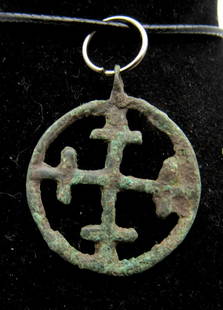The image depicts an antique circular pendant, resembling an archaeological find, hanging from a black string or wire against a dark, textured background. The pendant, centered in the photograph, is held by a silver O-ring and exhibits significant aging, with shades of green and brown rust intermixed with silver hues, giving it a weathered appearance, as though it has been submerged in water. The pendant features an intricate design with a cross-like symbol made of four T-shapes meeting at the center. The photograph, in full color and vertically oriented, captures the ancient, possibly Christian, artifact as it dangles in the stillness, shrouded by the blackness of the undefined setting.